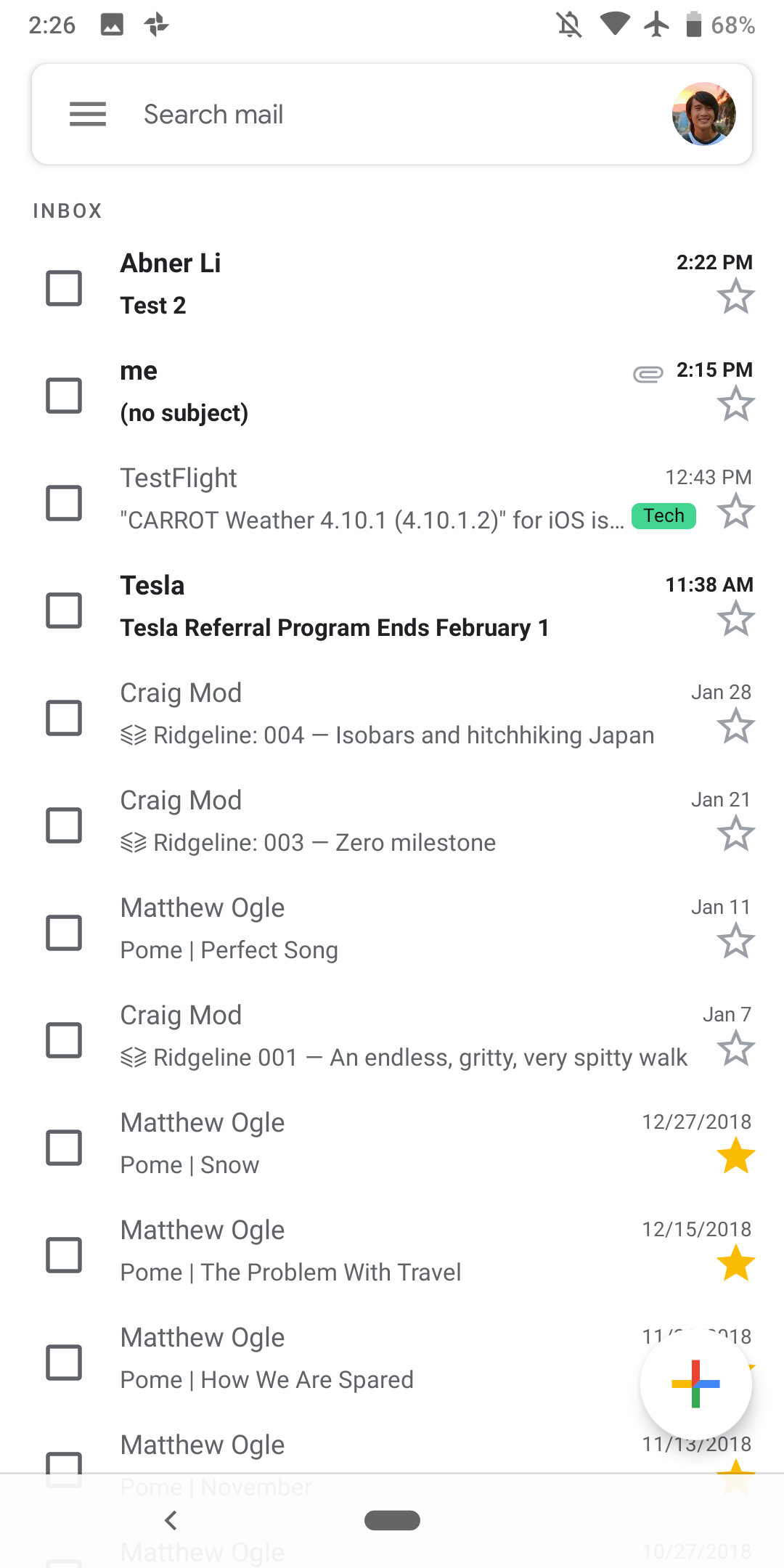A detailed screenshot of a mobile mail app displays various elements prominently. At the very top, the status bar indicates the current time as 2:26 PM, alongside two unidentified icons. To the right, icons for notifications off, Wi-Fi, and airplane mode are evident, along with a battery charge status showing 68%. Directly beneath the status bar, the search mail bar spans across the width of the screen, with a circular profile picture on the far right; the image is not clearly visible but hints at a person with short, dark hair.

The primary content of the screen is the inbox, showcasing emails in chronological order. The most recent email is from Avner Lee with the subject "test 2" received at 2:22 PM. Following this, the next email is a no-subject message sent by the user themselves at 2:15 PM. The third email, from Test Flight, concerns a version update labeled 'caret weather 4.10.1 (4.10.1.2) for iOS,' received at 12:43 PM. Tesla sent an email earlier at 11:38 AM. Two subsequent emails from Craig Mod are listed, followed by another from Matthew Ogle dated January 11th. Craig Mod appears again with an email dated January 7th. Further down, four emails from Matthew Ogle are marked with stars, indicating their importance. Alongside each email, a selection box on the left allows users to manage their emails efficiently.